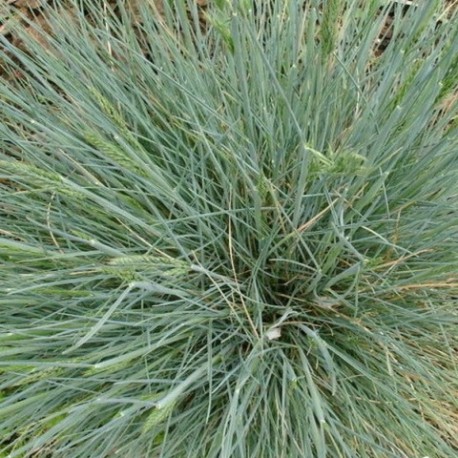The image is a close-up of a plot of overgrown, ankle-length grass, with a mixture of weeds and grass blades visible. The grass dominates the frame, standing in varying shades of green with some white, brown, and tan hues. The taller blades have darker green bulbs or seeds at their tips, adding texture and detail. Most of the grass strands are upright and spiky, while a few are bent over. The background is minimal, showing hints of brown—possibly rocks, dirt, or leaves—suggesting an outdoor setting in a forested or woodsy area during spring or summer. This patch of grass is the sole focus of the image, contributing to its artistic and somewhat wild appearance.